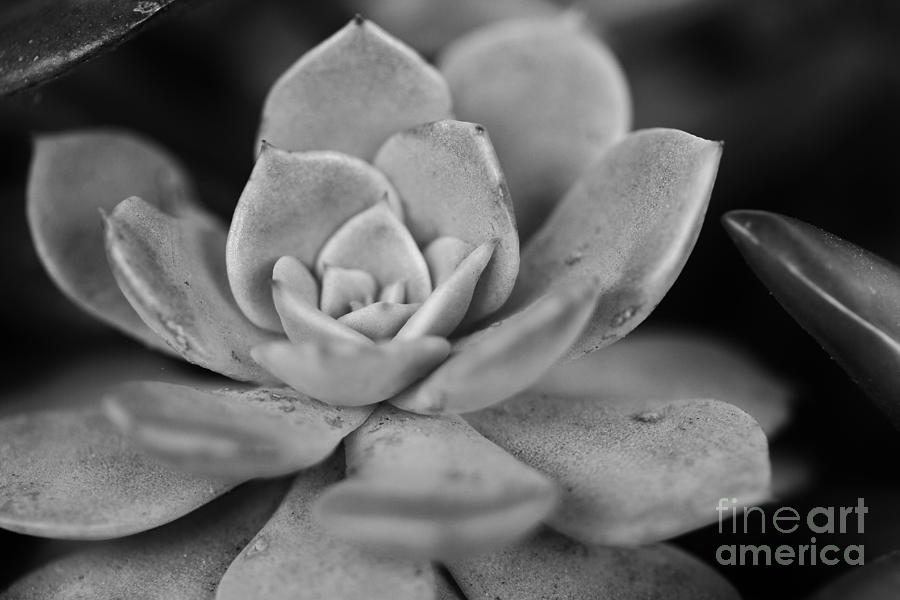This is a highly detailed and professional black and white close-up photograph of what appears to be a succulent or cactus. The image captures the plant’s intricate details, emphasizing its layered and pointy petals that open up gradually from a central bud. The succulent displays a range of grayish-white tones against a very dark, blurry background that adds depth and contrast to the composition. The photograph exhibits fine art qualities, with meticulous attention to shadow and light, presenting the plant almost as a sculptural piece. The lower right-hand corner of the image is marked with the words "Fine Art America," signifying its artistic value. Additionally, there are faint, darker shapes in the top left and right edges of the frame, which could be other plants or possibly objects, adding an element of mystery and further framing the main subject.